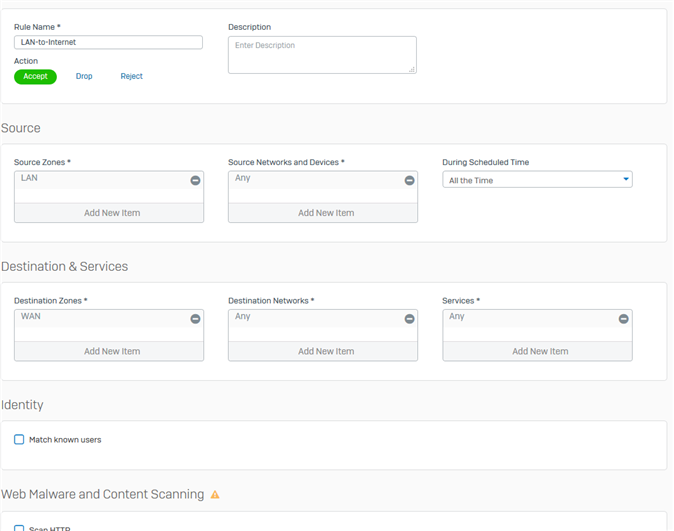The image is a screenshot from a utility webpage, likely for a software product designed for IT professionals. The incomplete view, missing both the header and footer, prevents identification of the company. The page's background is white, featuring an interface suggestive of server or network management.

At the top of the page, there is a section labeled "Rule Name" within a narrow rectangular box that reads "LAN to Internet." Directly below, the section labeled "Action" presents three options: a green rectangular button with rounded corners that says "Accept," flanked by "Drop" in blue text, and "Reject" in black text to the right.

Further down, the page is divided into three additional categories: "Source," "Destination," and "Services." Each of these categories includes three rectangular boxes, allowing the user to make necessary adjustments or selections. The interface is structured to facilitate configuration changes, typical for network or server management tasks.